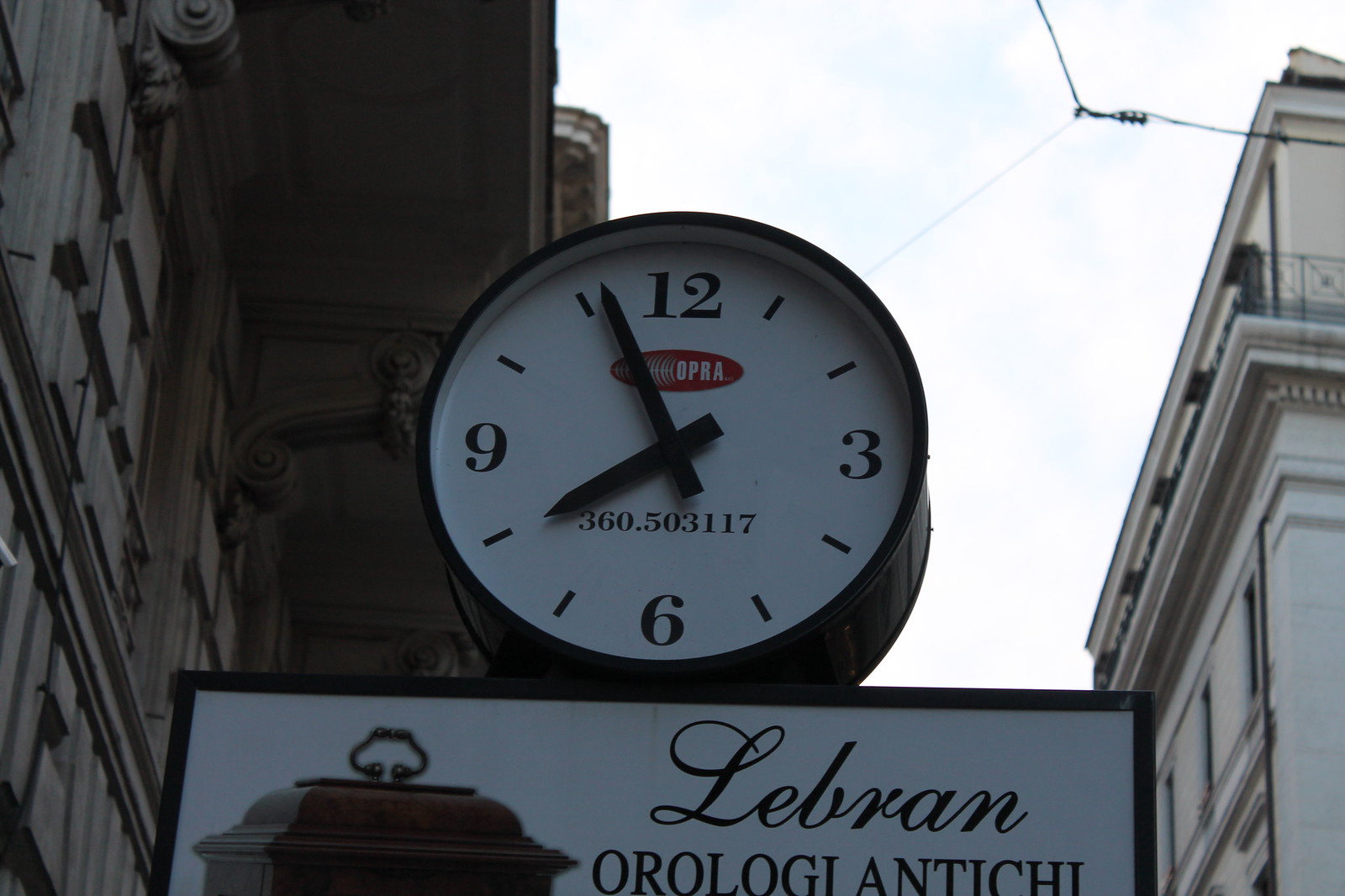The photograph captures a classic outdoor clock mounted atop a business sign. The clock has a dual-face design, although only one side is visible in the image. It features a traditional circular dial with prominent numerals at positions 12, 3, 6, and 9, while the remaining hours are denoted by simple hash marks. Curiously, the clock face also displays the numerals "360.503117," whose significance remains unclear. Below the clock, the business sign appears in black and white, prominently displaying the word "Lebron" alongside "Oro Logilantichi," which gives an Italian flair, suggesting a possible Italian heritage or theme of the business. The entire setup is attached to a building, and the angle of the photograph looks upward, emphasizing the stately presence of the clock and sign against the open sky.